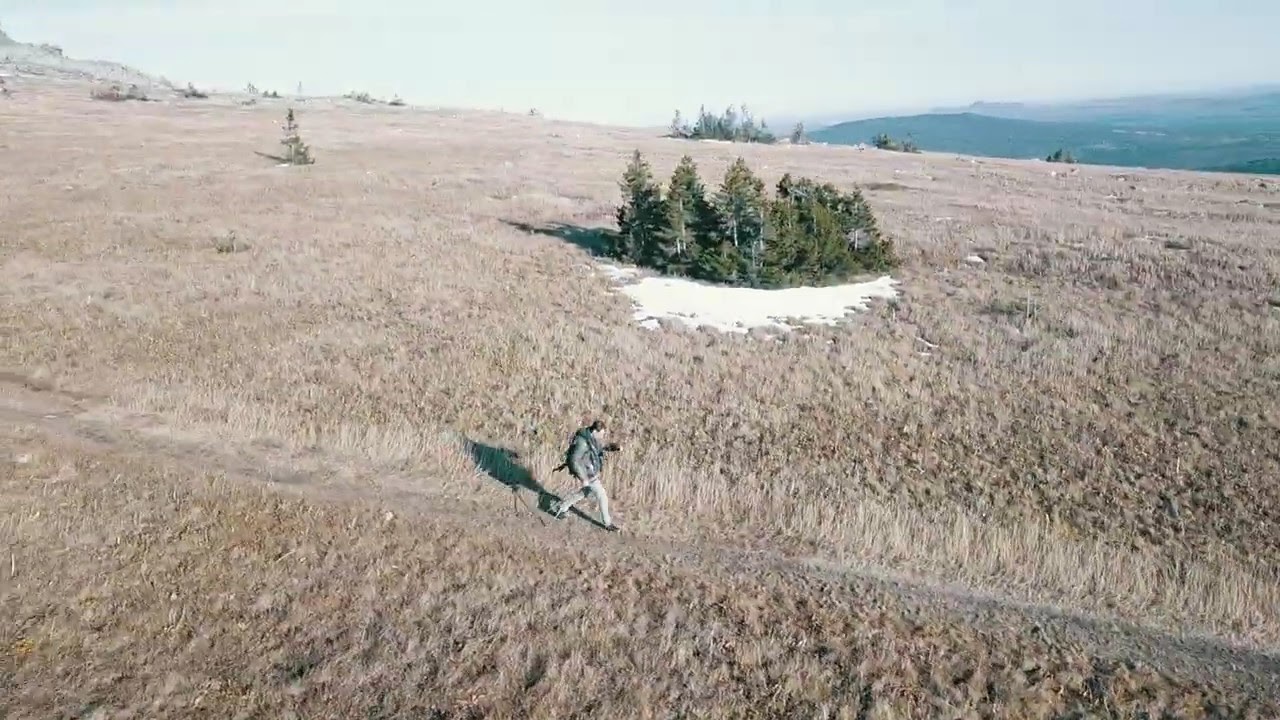A hiker, wearing light-colored pants, a green jacket, a backpack, and holding a walking stick, strides along a well-beaten trail on the flat summit of a mountain. His brown hair catches the light as he walks with one hand extended in front of him and his feet spaced far apart, each step casting a shadow behind him. The ground around him is a vast expanse of yellow-brown grass, contrasted by a distinct clump of evergreen trees at the center of the scene, their bases dusted with patches of white snow. In the backdrop, distant mountain ranges progress from lush green to muted gray, under a hazy, overcast sky. Despite parts of the photo being overexposed, the serene and rugged beauty of the landscape is clearly depicted.